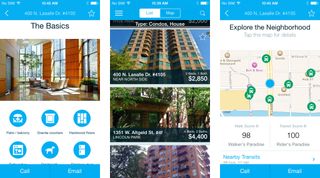The image is composed of three screenshots from a mobile application, likely related to a real-estate listing, presented on a white background with medium blue accents featuring extensively in headers and icons.

The first screenshot on the left, titled “The Basics,” displays an image of a luxurious apartment lobby. Beneath the image, several icons appear, presumably representing various amenities available within the building. At the bottom of this screen, there are buttons labeled "Call" and "Email" for easy contact options.

The center screenshot showcases a series of real-estate listings. It includes thumbnail images of different apartment buildings alongside their addresses and rental prices: $2,850, $4,400, and partially visible others. The format suggests a list where each entry provides a succinct overview of the property.

The third screenshot on the right is dedicated to the feature "Explore the Neighborhood." It presents a digital map dotted with icons likely indicating public transportation and other local services. There are two high "Walker's Score" values, 98 and 100, indicating excellent walkability, although the specific criteria for these scores are unclear. The same "Call" and "Email" buttons are consistently placed at the bottom of this screen as well.